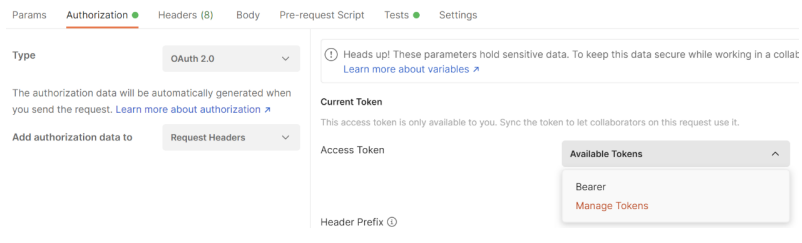This screenshot captures the settings interface of a web page or app, featuring a clean, white background. At the top of the interface is a navigation bar containing multiple clickable options. These options are displayed in gray font and include: "Params," "Authorization," "Headers (8)," "Body," "Pre-request Script," "Tests," and "Settings." 

The user has selected the "Authorization" tab, which appears in black font with a subtle red underline and a red circle next to it, indicating it's currently active. Additionally, the "Tests" tab also has a red circle next to it, suggesting there may be pending tests or notifications.

Beneath the navigation bar, the interface is divided into two white rectangular sections. The left section serves as the main configuration area. At the top, "Type" is displayed in gray font next to a drop-down menu currently set to "OAuth 2.0." Below that, a note in gray explains, "The authorization data will be automatically generated when you send the request," accompanied by a link in blue text labeled "Learn more about authorization."

Further down, another instruction in gray states, "Add authorization data to," beside another drop-down menu, which is labeled "Request Headers." 

To the right in the adjacent rectangle, a warning is presented in gray font, stating: "Heads up! These parameters hold sensitive data. To keep the data secure while working in a collect..." The warning text appears truncated, indicating the presence of additional information not fully visible in the screenshot.

This detailed description encapsulates the essential elements and functionalities displayed within the settings interface, highlighting the current focus on authorization settings and relevant user guidance.